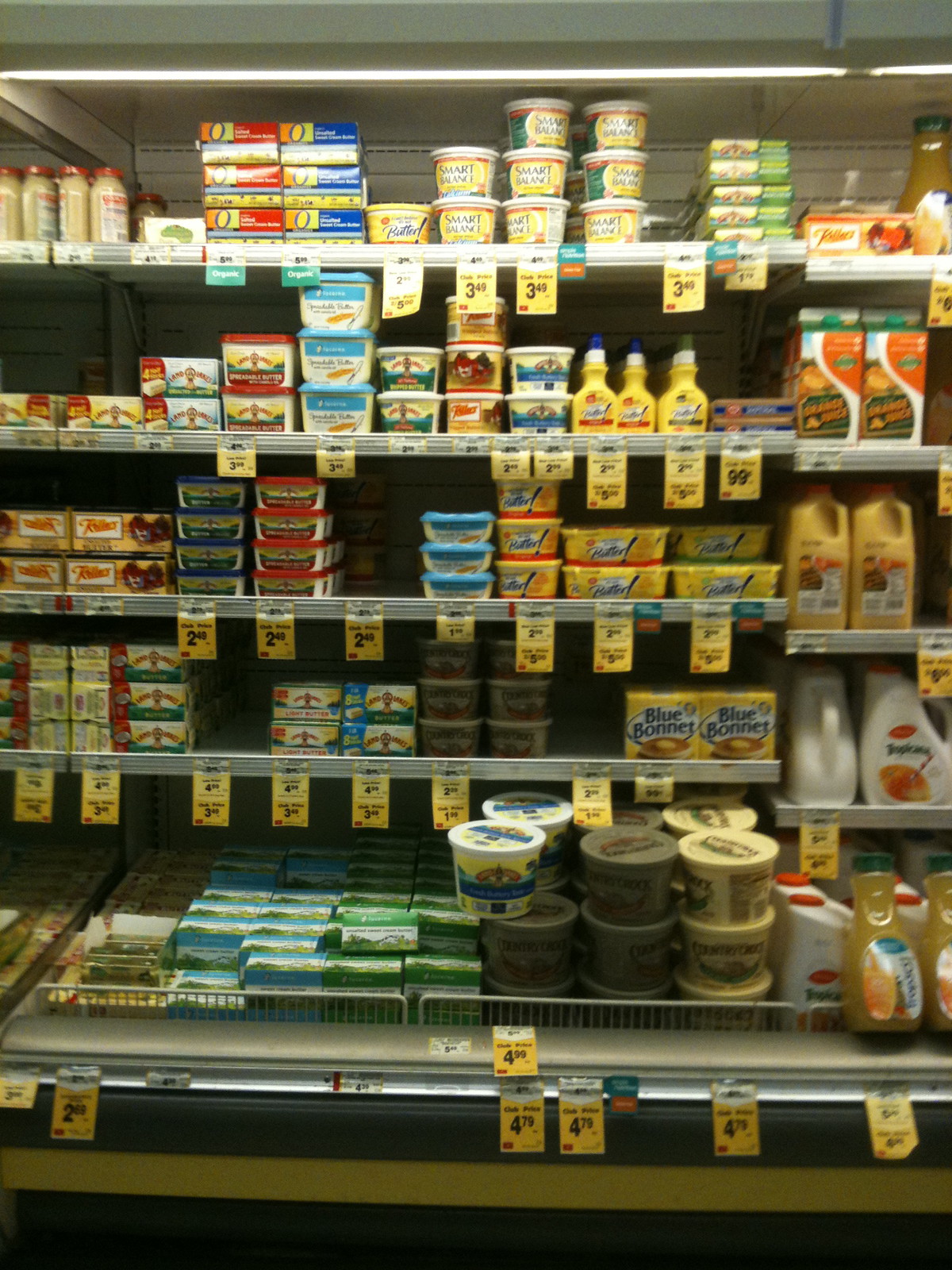The image depicts a well-lit grocery store aisle, specifically the cold dairy section, showcasing a variety of butter and margarine products neatly organized on shelves. The top rows are filled with an assortment of brands including Land O'Lakes, Smart Balance, I Can't Believe It's Not Butter, and Challenge Butter, along with some store brands, and items like Imperial Butter. The shelves feature both tubs and boxed sticks of butter in assorted colors such as yellow, green, and blue. On the right side of the image, shelves transition from dairy products to various orange juice brands, including Tropicana and Florida’s Natural, adding a pop of orange to the scene. The items are all priced from 99 cents to over five dollars, with yellow price tags beneath each product. The aisle is illuminated by bright fluorescent lighting, enhancing the vibrant colors of the packaging and maintaining a cool environment for the dairy products.